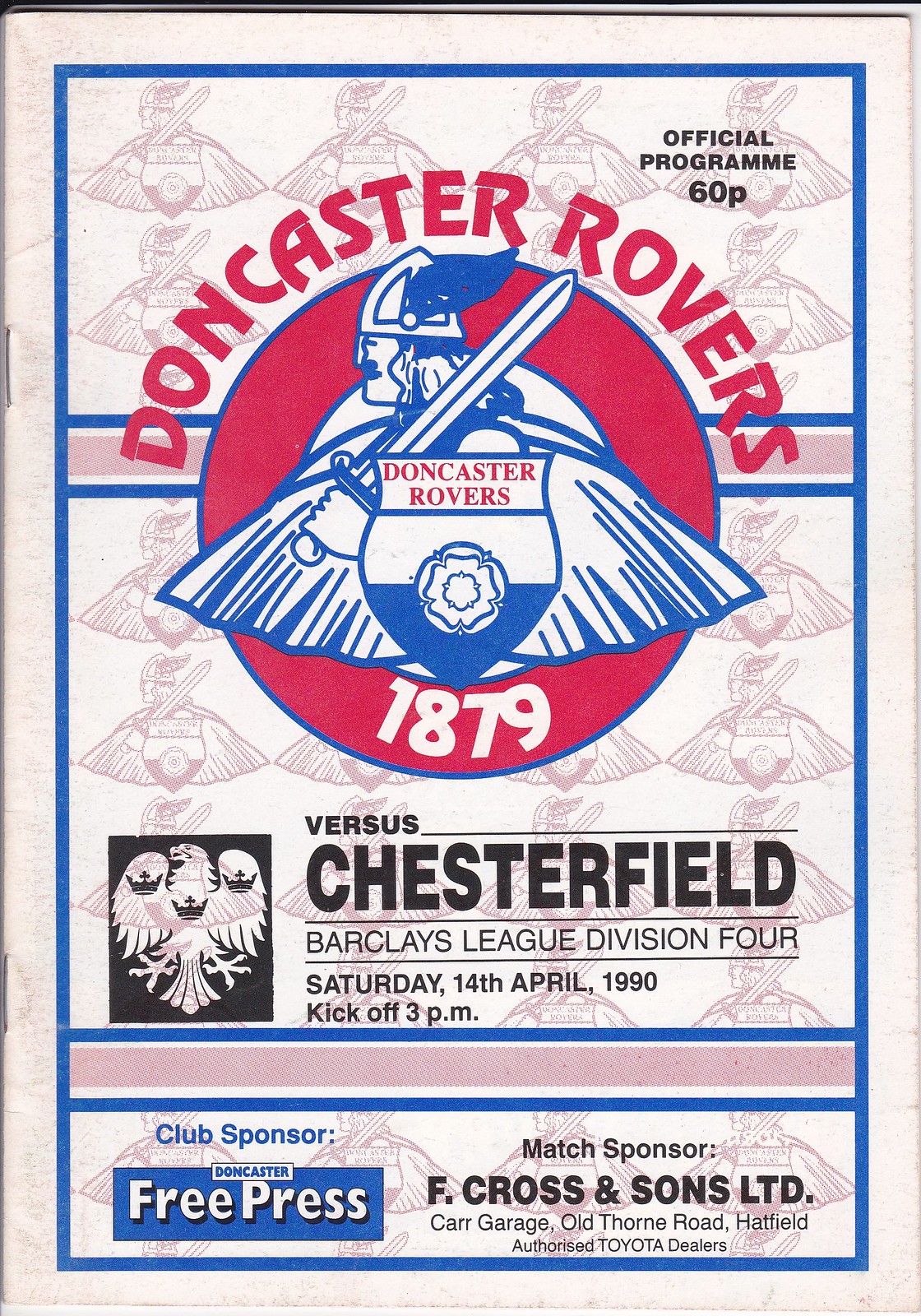This is a detailed close-up photograph of an official program for a Barclays League Division 4 football match between Doncaster Rovers and Chesterfield, held on Saturday, April 14, 1990, with a kickoff time of 3 p.m. The program, priced at 60 pence, features a stapled binding, indicating it is a small booklet. The overall design employs a vintage aesthetic with a tan background and red, white, and blue color scheme, which gives it a nostalgic feel. Dominating the center of the cover are the words "Doncaster Rovers" in bold red text, arching around a circular emblem. This emblem showcases a Viking with a helmet, feather, and sword, outlined in blue against a white backdrop, symbolizing the club's logo. Below this, the founding year "1879" is prominently displayed. Further down, it states "versus Chesterfield" and provides the match details such as the league, date, and time. The background of the entire program subtly features the Viking emblem as well. In the top right corner, it reads "Official Program 60p" in black text. The club sponsor, Doncaster Free Press, and the match sponsor, Cross and Sons Limited Car Garage on Old Thorn Road, Hatfield, authorized Toyota dealers, are also mentioned, reflecting the local support and endorsement for the event.